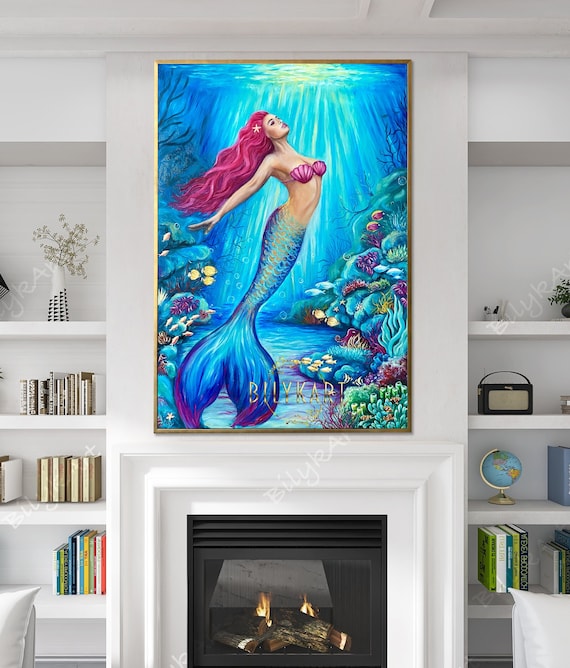The image depicts a cozy living room featuring a dominant black fireplace with a few pieces of wood burning warmly, framed by a neat, white rectangular mantle. Above the fireplace, a striking gold-framed painting captures attention: it’s an underwater scene with a mermaid, characterized by her long pink and purplish hair, pink seashells, and a blue and pink scaled tail, all illuminated by rays of sunlight filtering through the water. This vivid artwork, with a blue background, has a translucent white watermark reading "Billy Cart," while the watermark on the painting itself is a distinguished gold logo.

Flanking the fireplace are two four-tiered white bookcases filled with a mix of books, a small globe, vases, and various home decor items, adding charm and personality to the room. The walls and ceiling are also white, enhancing the room’s bright and airy atmosphere, making it a visually pleasing and inviting space.